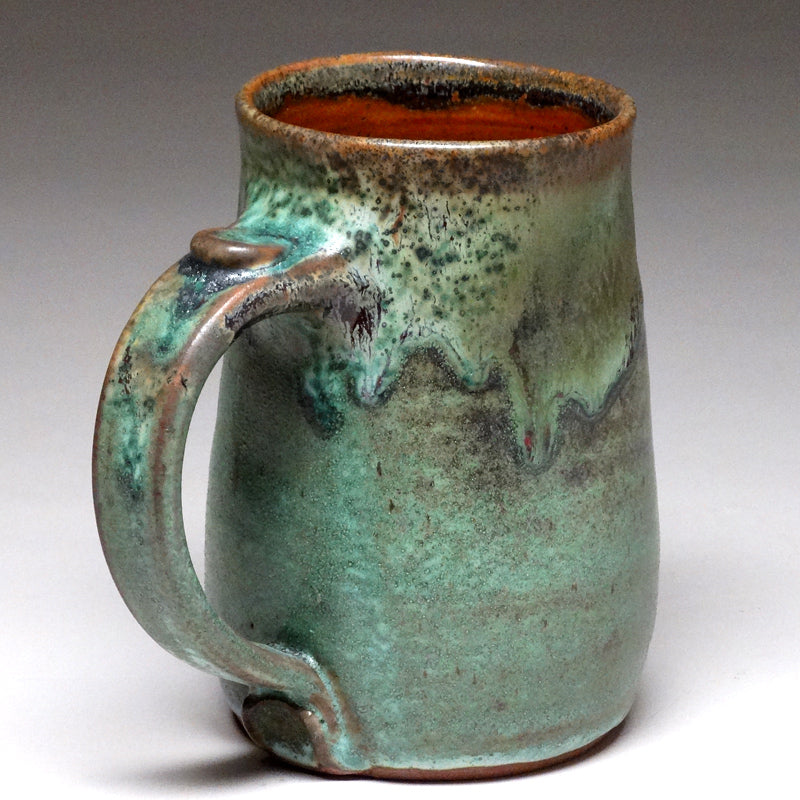This color photograph features an intriguing ceramic mug, positioned with its handle to the left against a white and gray background. The mug, made of clay, shows signs of being older and somewhat worn, but it retains a glossy finish on the exterior. The handle, with a small nub on top designed for thumb placement, extends from the bottom of the cup up to about four-fifths of its height. The mug is glazed with a striking greenish-grey, almost metallic, color. This glaze appears to have run down from the top, creating a visually appealing drip effect. 

The rim and parts of the handle exhibit a speckled black and brown finish, with hints of wear that add a rustic charm. Inside, the mug reveals a light, rich brown hue, contrasting with its more complex exterior. Additionally, small dark specks and the overall combination of black and green tones give the effect of an aged, yet artistically crafted piece. This beautifully captured mug rests on what seems to be a white table, with a subtle shadow adding depth to the composition.